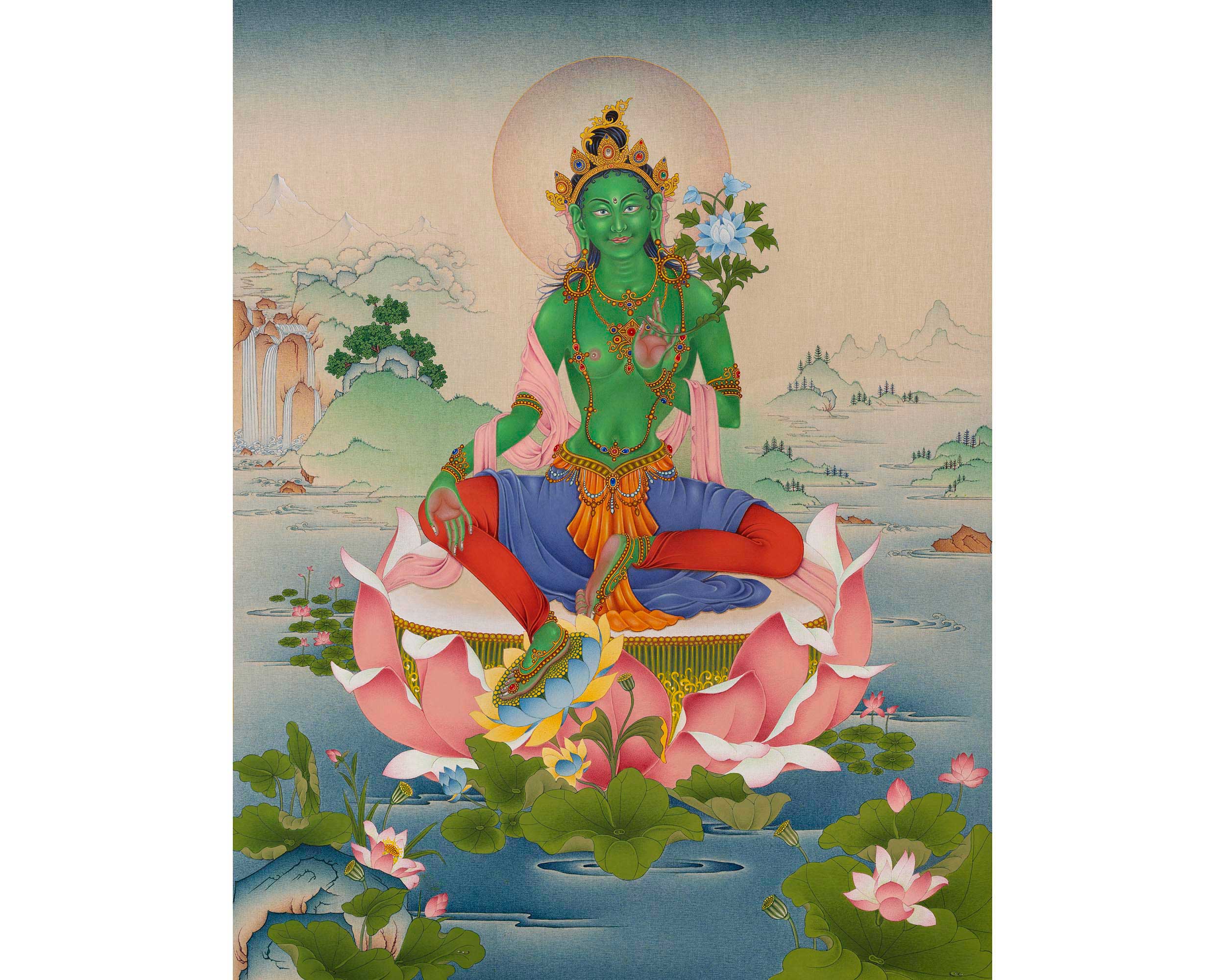This detailed artwork features a Hindu or Buddhist deity, likely a goddess, depicted with a rich blend of vibrant colors and intricate details. The central figure, distinctly characterized by her green skin, is adorned with a gold crown encrusted with red, white, and blue stones, and a pink shawl draped elegantly around her arms. She wears a navy skirt, red leggings, and green and red footwear, with an orange belt cinched around her waist. Her pose is serene, with one hand raised by her chest and the other resting near her knee, as she sits cross-legged on a large, pink lotus flower floating in a tranquil blue pond.

The background merges elements of natural beauty and celestial symbolism: a radiant disk, possibly representing the sun or moon, frames her head with a light pink hue, while behind her, the sky transitions into a pinkish tint reflecting either dawn or dusk. The scene expands to reveal a waterfall, rock structures, lush greenery, and distant mountains, adding depth and tranquility to the image. The pond is adorned with green lily pads, some bearing pink blossoms, adding to the serene, almost sacred ambiance of the artwork.